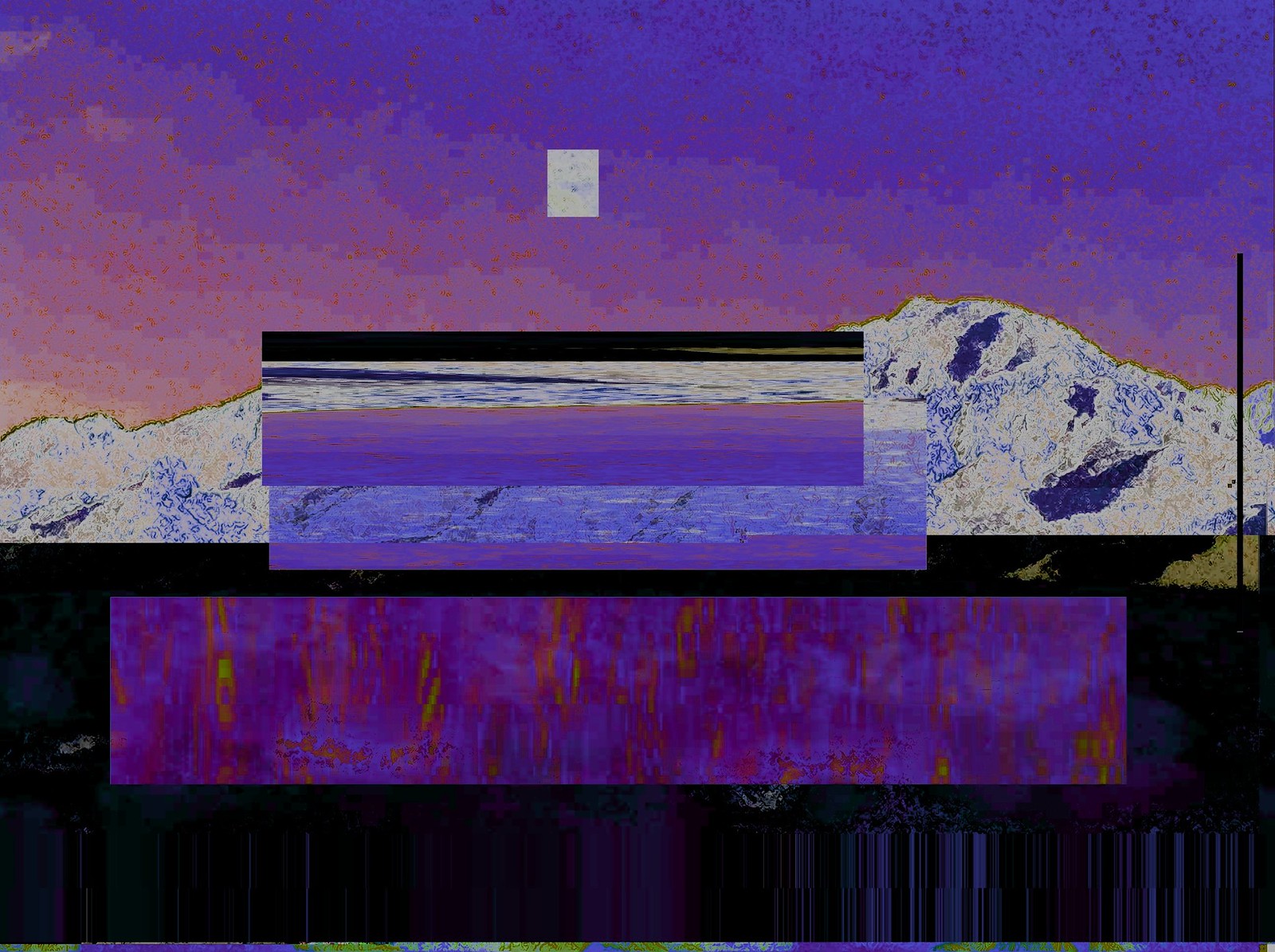The image is an abstract, computer-generated painting dominated by shades of purple. It features a series of visually striking elements. At the top, the sky transitions from a dark purple at the very top, becoming lighter as it reaches the mountainous region. The sky exhibits water-like brush strokes and contains a square, white-colored moon. Immediately below this sky, there are glacier-like formations on either side of the image, characterized by alternating patterns of glacial ice and purple water bodies arranged from top to bottom.

Amidst these formations, scattered red speckles add an additional layer of texture across the painting. In the center, there is a juxtaposition of colors including blues, pinks, and purples across rectangular areas, contributing to the painting's abstract quality.

Dominating the lower section, there is a substantial dark band—almost black but interspersed with shades of green, purple, and white. Centrally positioned is a large, distinctive purple bar featuring reddish lines, reminiscent of wood grain or tiger stripes. Above this bar, overlapping rectangles exhibit blended hues of violet, blue, and white, further enhancing the abstract and layered aesthetic.